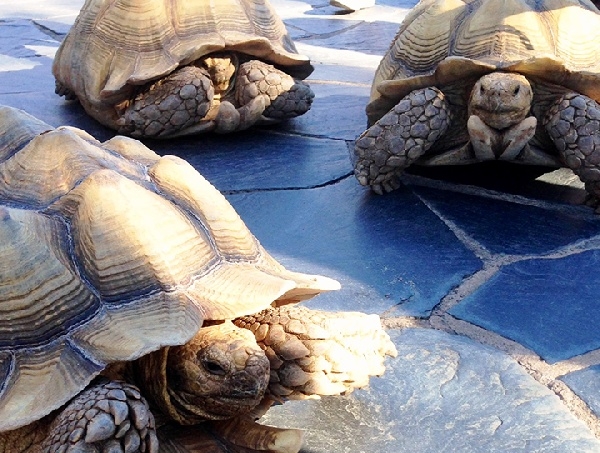The image captures a group of three large tortoises on a gray, man-made stone floor, basking in natural sunlight. The ground consists of gray stones with visible grout lines and speckles of dirt, suggesting an outdoor setting, possibly a controlled environment like a zoo. The tortoises, characterized by their rough, scaly, and predominantly green skin, exhibit varying shades of brown and gray, especially on their faces and limbs. Their shells are large, with a distinctive tan and black groove pattern that looks particularly clean and shiny, as if recently washed. In the background, one tortoise partially retreats into its shell while the others roam and explore. A faint shadow of a figure looms over one of the tortoises, and a white tennis shoe with black trimmings is barely visible in the back of the scene, providing a hint of human presence.